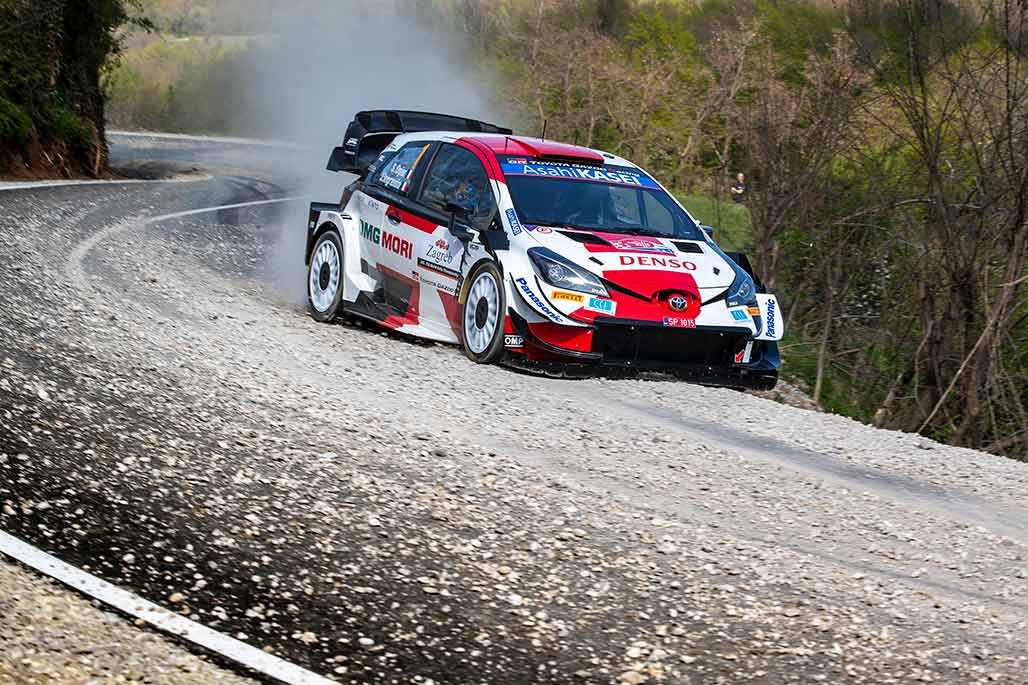This is a detailed photograph of a white race car with prominent red and navy accents, featuring various sponsorship logos such as "Asahi Kasai" on the windshield, "Denso" on the front bumper, and "OMG Mori" along the left side. The car appears to be veering off a winding, asphalt road, partially resting on the shoulder, surrounded by a plume of white smoke trailing from its rear. The road is covered in small rocks and debris, with visible white lane markings. The setting includes dense trees, bushes, and shrubbery alongside a slight drop-off from the road, contributing to the image of a secluded, challenging race track. Additional details such as a large black piece hanging off the back and the mix of dirt and pollen on the road's surface add to the sense of a dynamic and gritty racing environment.